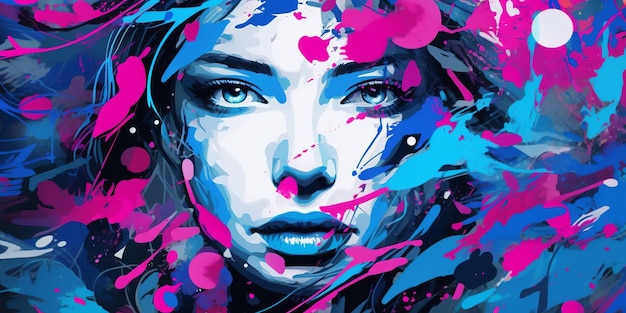The illustration is a horizontally placed, rectangular painting dominated by hues of purple and blue. At the center of the image, a woman's face stares directly at the viewer with striking blue eyes, accentuated by blue highlights around them. Her blue hair frames her face, which is noticeably light with a white center. Dark, almost black eyebrows and blue lips, highlighted further by a layer of blue lipstick, emphasize the bold color scheme. Her face is surrounded by abstract designs featuring leaf-like or spotted patterns in pink and blue, interspersed with additional lines and spots of green paint. These vibrant colors and smeared paint strokes encase her face, adding a layer of abstract complexity and a touch of mystery, making the overall style evocative of a cartoon or animated painting.